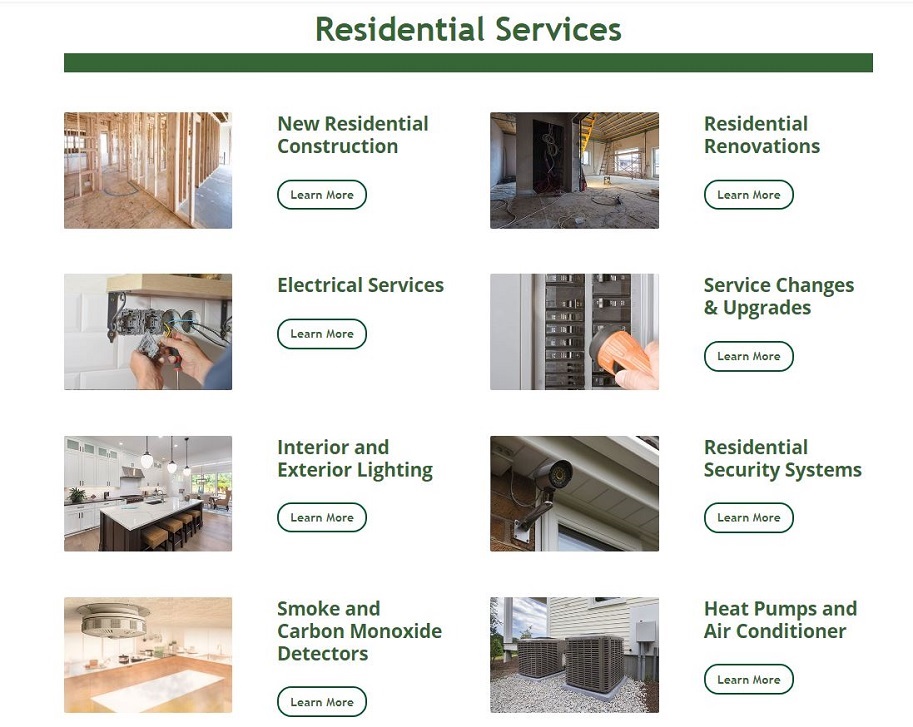The image showcases a professionally designed webpage or advertisement with a clean, white background. At the top, there's a green banner prominently displaying "Residential Services" in bold, green text. Below the header, various images illustrate the range of services offered.

1. **New Residential Construction**: An image showcases the early stages of a home build, with wooden frames being erected. A green "Learn More" button invites viewers to explore this service in detail.

2. **Residential Renovations**: Another visual depiction shows a developed neighborhood with homes either under construction or being renovated. This section also contains a "Learn More" hyperlink.

3. **Electrical Services**: A photograph captures a technician working on an electrical box, indicating services like changes and upgrades. Another image features an electrical panel with multiple switches, emphasizing the range of electrical solutions available.

4. **Interior and Exterior Lighting**: A beautifully lit, modern kitchen highlights the company's expertise in both interior and exterior lighting installations.

5. **Residential Security Systems**: An image of a mounted security camera represents the service offerings in home security, including installation of smoke and carbon monoxide detectors, as well as heat pumps and air conditioners.

Each section is accompanied by a detailed, corresponding image, enhancing the visual appeal and providing a clear understanding of the diverse residential services offered.